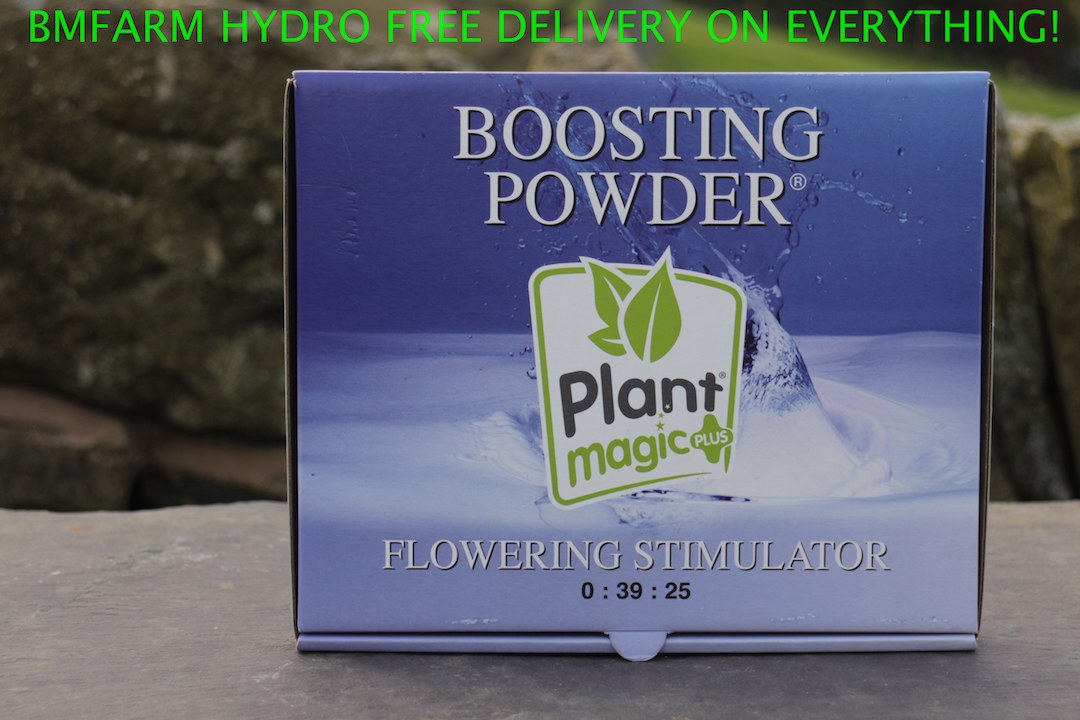This image depicts a nearly square, blue cardboard box placed on a textured surface, which appears to be rocks, suggesting that it might be either outdoors or in a rustic setting. The box prominently features a white square in the center, showcasing a logo with two green leaves and the text "Plant Magic Plus." Above the logo, in white letters, is the phrase "Boosting Powder," and below it, also in white letters, is "Flowering Stimulator," followed by "0:39:25" in black letters. The background of the box illustrates water droplets impacting a water surface, creating a splash effect. At the very top of the box, in green capital letters, is the text "BM Farm Hydro Free Delivery on Everything." The primary colors in the image include blue, white, green, and black, contributing to the overall vibrant and eye-catching design of the package.